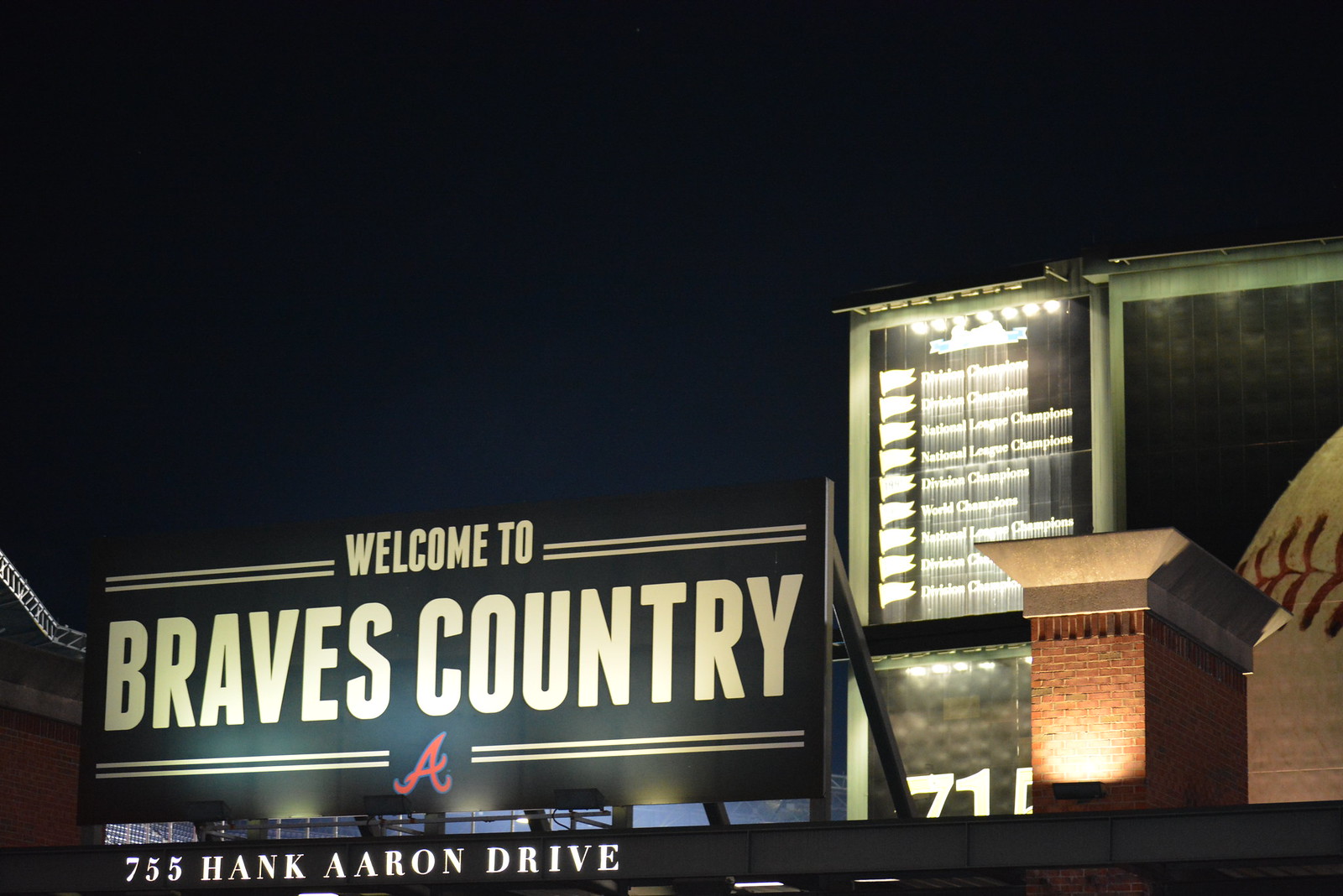The photograph, taken at night with a black sky dominating the top two-thirds of the image, captures the entrance of the Atlanta Braves stadium. The scene features a prominent overhead sign that warmly welcomes visitors with the text "Welcome to Braves Country" in large white illuminated letters. The "Welcome to" part has two horizontal lines extending from it, and centrally beneath it is the emblematic red Atlanta "A," styled in cursive and outlined in blue, with additional horizontal lines extending from the letter. To the right, there's a tan-colored wall displaying a somewhat blurry inscription detailing the Braves’ various championship titles like "World Champions" and "Division Champions." Below part of this text, the numbers "7-1" of an address are visible. An imposing brick column with a white top adds to the architectural detail in the foreground. Situated prominently is a clearly readable black sign with "755 Hank Aaron Drive" in all caps, illuminated and likely affixed to an overhang, marking the historic address. The photograph captures the night-time ambiance of the stadium entrance, with every detail contributing to the grand sense of place and history.